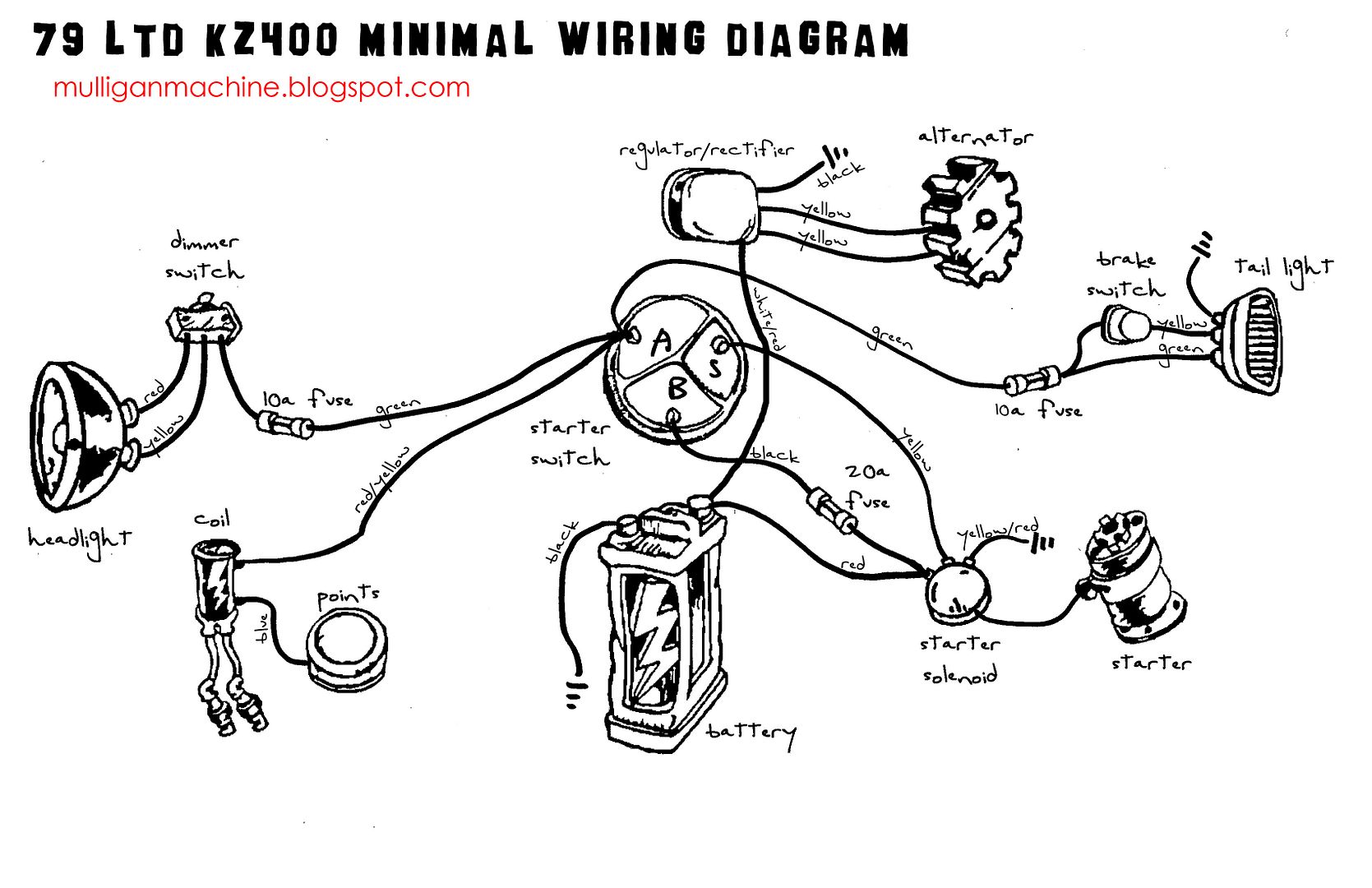The image titled "79 LTD K2400 Minimal Wiring Diagrams in Black Forms," prominently displays a complex, hand-drawn diagram within a horizontal rectangle. Below the title, in red text, the website "mulliganmachine.blogspot.com" is indicated. The black-and-white drawing intricately maps out the wiring connections between various automotive components.

On the left, a headlight is depicted, connected by two wires to a dimmer switch, which subsequently connects to a 10A fuse and then to a central starter switch. The starter switch, labeled with "A," "B," and "S," is the focal point of the diagram, with numerous connections radiating from it, resembling the limbs of an octopus.

Nearby, a coil and point assembly is connected to the starter switch, alongside a large battery positioned at the center bottom. The battery, marked with a lightning bolt, has multiple cables leading to ground, a regulator rectifier at the top of the image, and a starter solenoid on the right side. The starter solenoid, in turn, disperses five wires to various elements, including the starter itself, a 20A fuse, and directly to the "S" terminal on the starter switch.

Additionally, a taillight occupies the upper right section, with its three wires connecting to ground, a brake switch, and a 10A fuse, which then routes to the "A" port of the starter switch. Above the taillight, the alternator sits to the right of the regulator rectifier, with two wires connecting them and an extra wire leading to a ground point.

This meticulous layout effectively illustrates the minimal but essential connections required in the diagram, detailing each component and its interlinked pathways with precision.